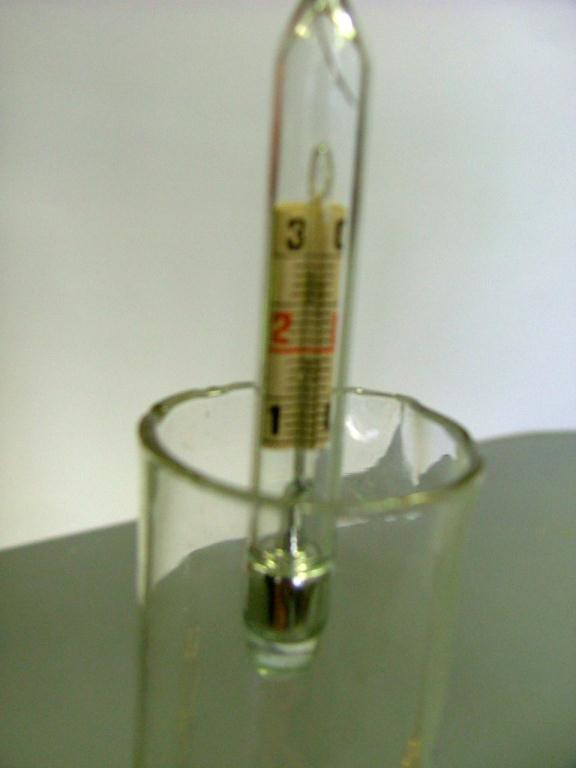In this rectangular, vintage-style photograph, a long, vertical image captures a scene with a distinct grainy texture. Set against a dark gray table or countertop, there is a clear, cylindrical glass tumbler reminiscent of laboratory equipment. Inside the tumbler, a specialized thermometer is prominently featured. Unlike typical household thermometers, this one is oblong and clear, with a white background for its measurement scale. The numbers "3", "2", and "1" are marked sequentially from top to bottom, with "3" in black, "2" in red, and "1" in black text. The image is notably grainy, causing the glass tumbler and the thermometer to appear slightly blurred. Inside the thermometer, the presence of a clear liquid can be discerned, and it is topped with a shiny metal tip resembling the base of a light bulb. Despite the intricate detailing, the graininess of the photograph makes it difficult to read the exact temperature measurement on the thermometer.